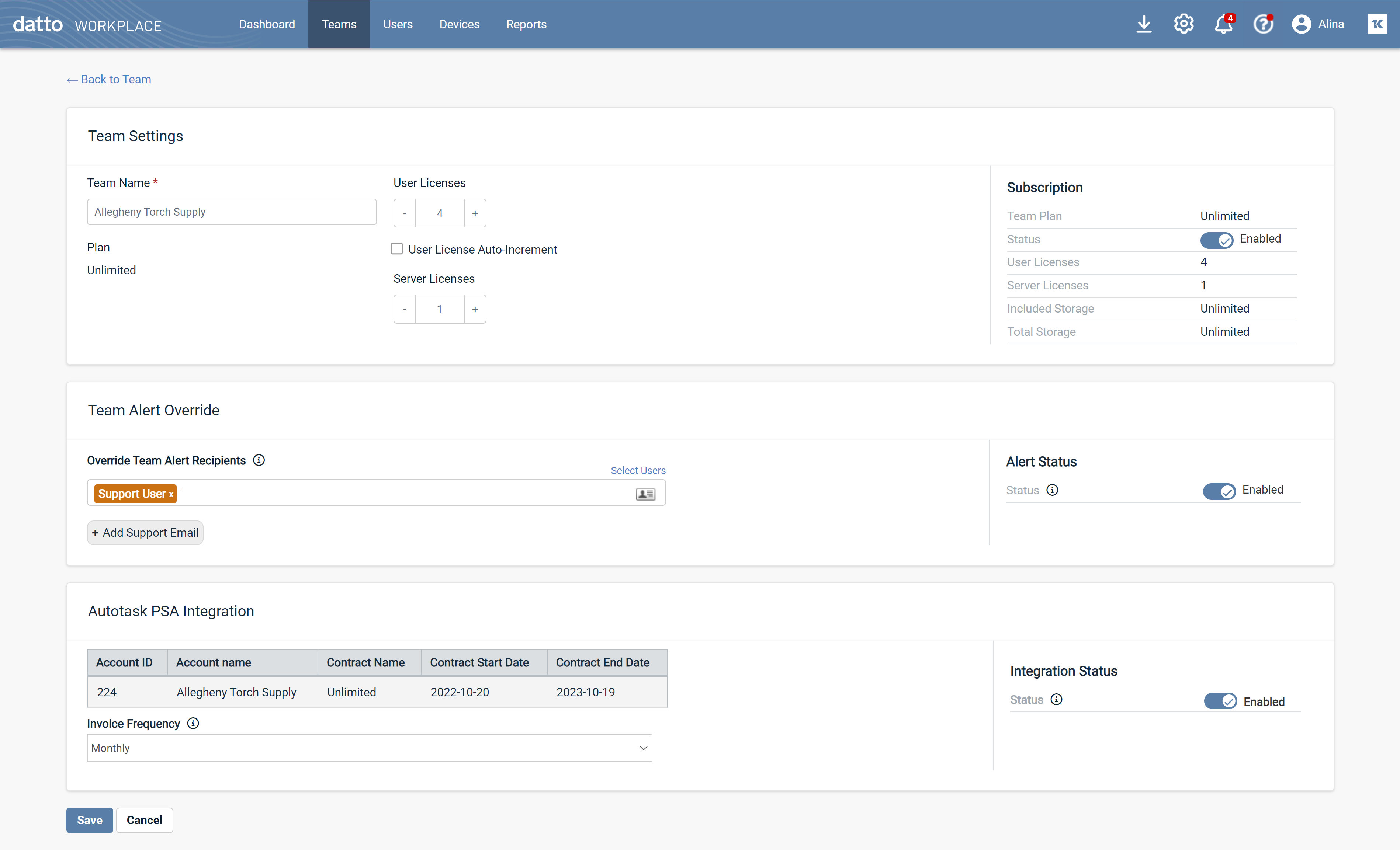This is a detailed screenshot of a website named "Datto Workplace," resembling a Slack-like platform for online collaboration. Capturing the entire website interface — excluding the address bar — the image shows various interactive elements designed to facilitate communication and teamwork.

On the top left, the website's name "Datto Workplace" is prominently displayed. Adjacent to the name, a menu bar features several tabs for navigating different sections: "Dashboard," "Teams," "Users," "Devices," and "Reports." The "Teams" tab is highlighted, indicating it's the currently active section.

On the top right corner, there are several intuitive icons for additional functionalities: a gear symbol for settings, a notification bell, a download icon, and a question mark for help. Both the notification bell and question mark icons have red numerical indicators, suggesting there are unread notifications and help tips awaiting the user's attention.

Below the navigation bar, the content area appears to display settings for different teams. You can see fields and options for configuring the team name, plan, team alert override, and similar settings, allowing users to customize their teams according to their specific needs. This comprehensive view underscores Datto Workplace's role as a collaborative online workspace.